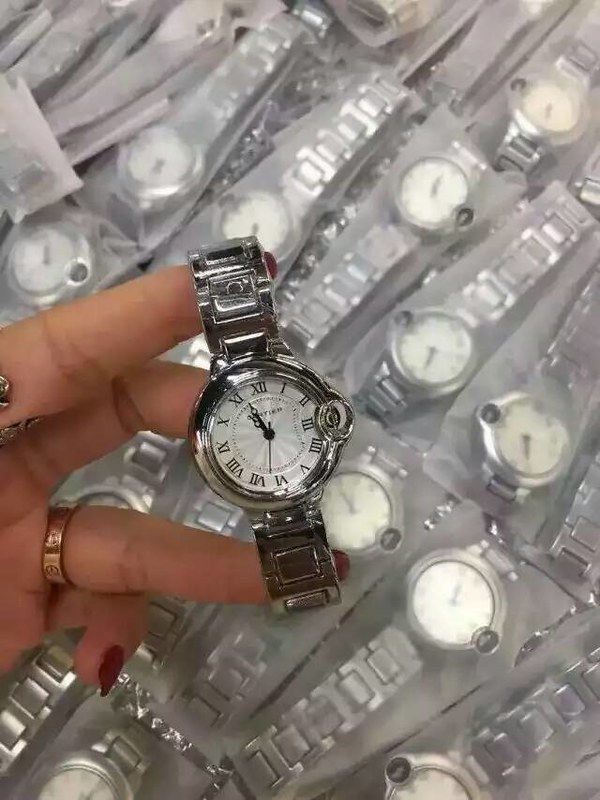A detailed image showcases a multitude of identical silver-toned watches sealed in clear plastic bags. These watches feature small, white faces adorned with black Roman numerals from 1 to 12, with a slight curve at the 3. The elegant design includes thin, long second hands alongside thicker hour and minute hands, each having a hollow circle at the tip. Above the array of packaged watches, a woman's left hand, with distinctively red acrylic nails, holds one watch outside its packaging. She has the watch looped between her ring and forefinger, revealing its intricate design. She wears a ring with a unique dip on her index finger, and a gold or copper ring on her ring finger. The displayed watch's silver wristband and edging around the face glimmer, accentuating its classic appearance. The woman's demonstration seems to highlight the watch's features, possibly for a sales purpose.